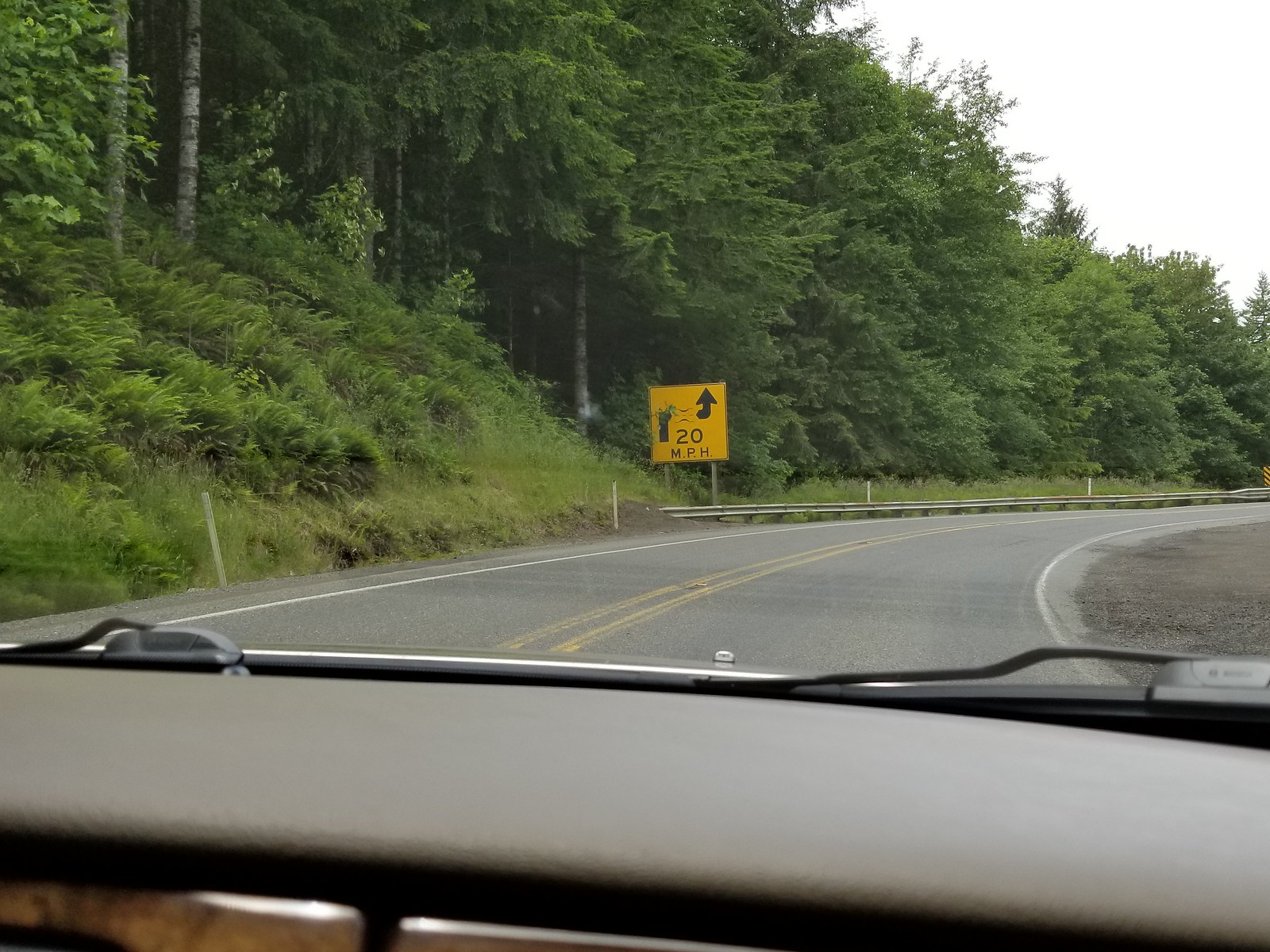This dash camera photograph captures a serene two-lane road flanked by lush green trees under a clear, white sky. The bottom portion of the image shows the gray dashboard and windshield wipers of the vehicle, with the road stretching ahead and then curving out of sight to the right. A double yellow line runs down the center of the road, providing a guideline for the lanes. On the right side of the road is a small gravel loop, while a guardrail borders the opposite side. Centrally positioned within the image is a yellow road sign indicating a speed limit of 20 MPH, topped with a partially obscured, squiggly arrow, suggesting a winding road ahead. A vertical black bar appears on the left side of the sign, contrasting with the arrow on the right. The leafy canopy of trees envelops the scene, creating a picturesque and peaceful driving environment.